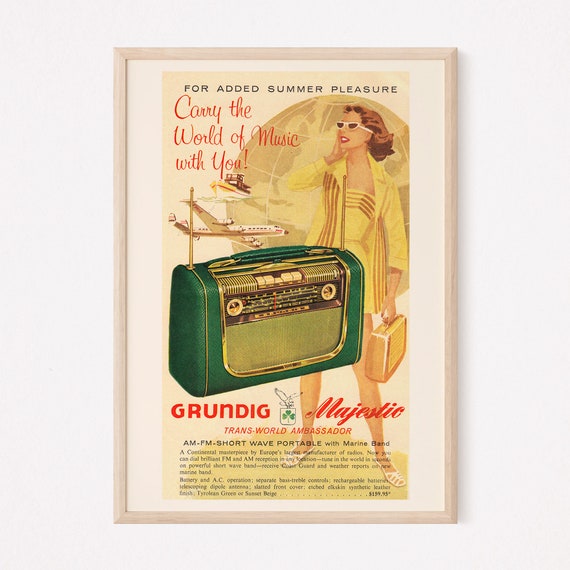The image is a detailed photograph of a retro travel advertisement poster, housed in a light brown wooden frame, mounted on a light gray wall. The overall photograph is square-shaped, but the poster within it is rectangular, with the left and right sides twice as long as the top and bottom. The poster prominently features a large green vintage radio with gold buttons and trim. Above the radio, in gray text, it reads, "For added summer pleasure." Further down, in a vibrant red font, the text proclaims, "Carry the world of music with you."

Dominating the background is a stylized illustration of a woman dressed in a yellow dress with red stripes and a matching yellow coat. She has wavy brown hair and is accessorized with white sunglasses. The woman is holding a yellow suitcase and is set against a backdrop featuring a globe. Complementing the travel theme, an airplane and a ship are depicted towards the left side of the poster. Below the woman and the radio, the text, "Grundig Majestic Trans World Ambassador, AM, FM, shortwave portable with marine band," is displayed. The poster concludes with the tagline, "A continental masterpiece by Europe's finest," highlighting the grandiose and global appeal of the product.